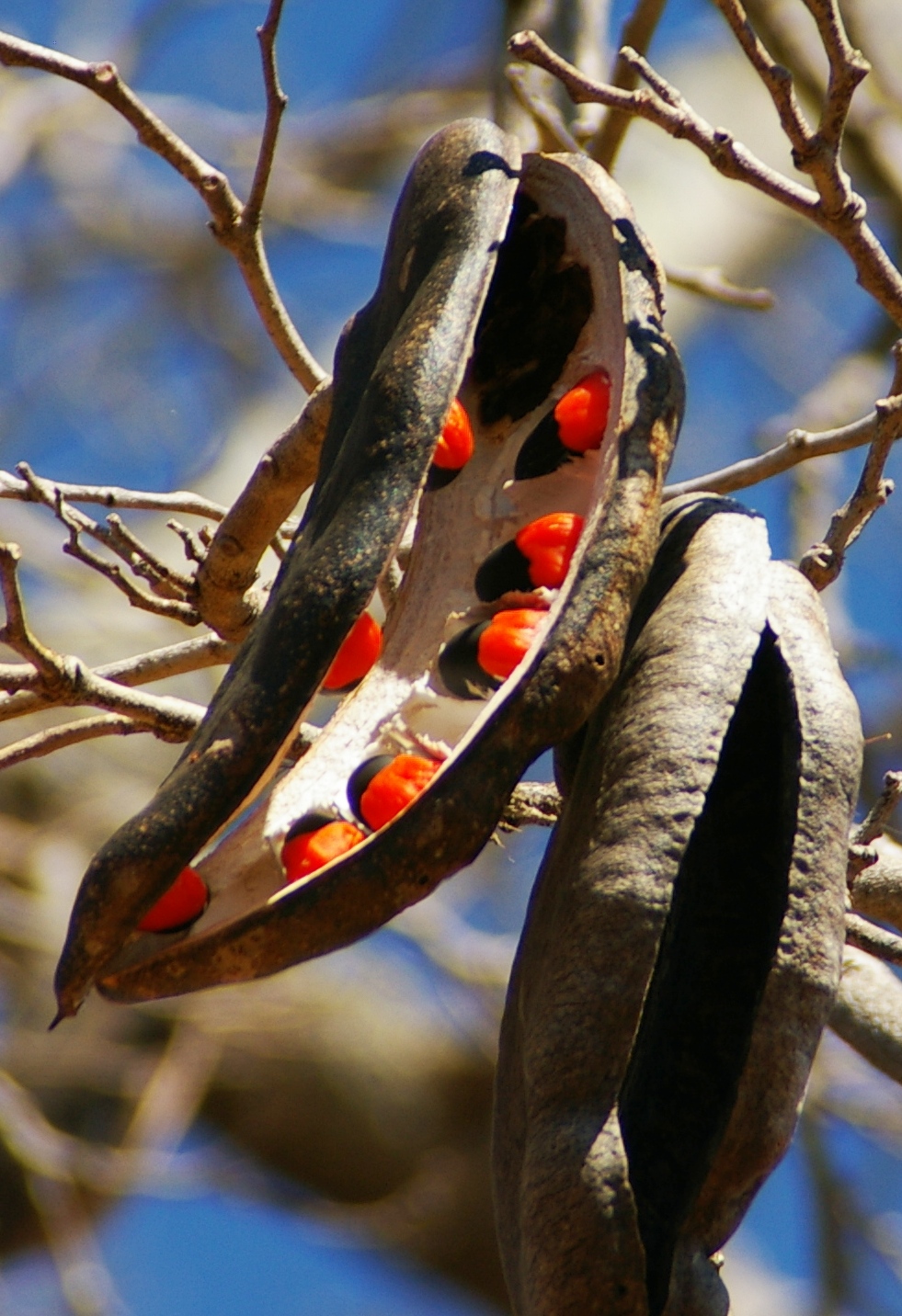In this professional photo, we observe a sunlit scene featuring a unique fruit hanging from a tree. The central focus showcases two elongated, brown fruits that have split open, exposing their interiors. The outer shells curl slightly and their surfaces are aged. The bright sunlight highlights the inner parts of one of the fruits, revealing a striking contrast between the white interior and the vivid, glowing red berries nestled within. Surrounding the fruits, we see a web of small, intertwined branches set against a blurred backdrop that hints at a clear blue sky and possibly some trees. The blend of natural colors including shades of brown, red, orange, blue, and white, adds to the captivating details of the outdoor setting captured on a sunny day.